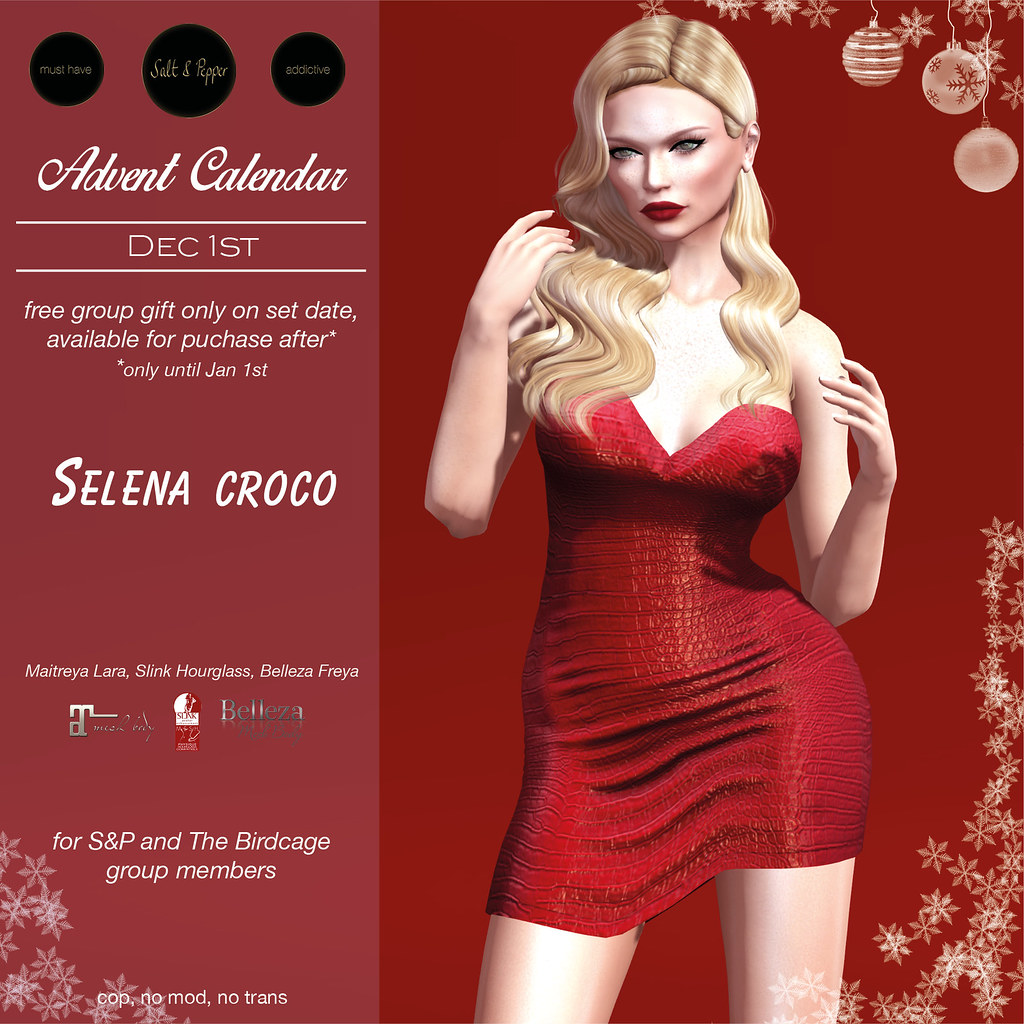The poster is a festive Christmas-themed advertisement, predominantly featuring a vibrant red color scheme. The left side presents a striking animation of a blonde woman in a short, tight red dress that highlights her chest-length, curly hair. The background behind her is solid red, creating a captivating contrast with her bright skin. She appears to be raising her arms, perhaps to touch her hair, which cascades down both sides of her head.

Christmas decorations adorn the poster, with white ornaments hanging from the top right corner and a light snowfall effect in the lower right corner. A slightly softer red bar runs down the left side of the image, with the text "Advent Calendar" in bold white letters. Below this, "December 1st" marks the beginning of the calendar, followed by the message: "Free group gift only on set date, available for purchase after. Only until January 1st."

Several sponsor names are listed, including "Selina Kroko," prominently displayed alongside "for S&P and the Birdcage group members." The poster also features three small black circles with "Must Have," "Salt and Pepper," and "Addictive" inscribed within them, emphasizing the allure and exclusivity of the event.